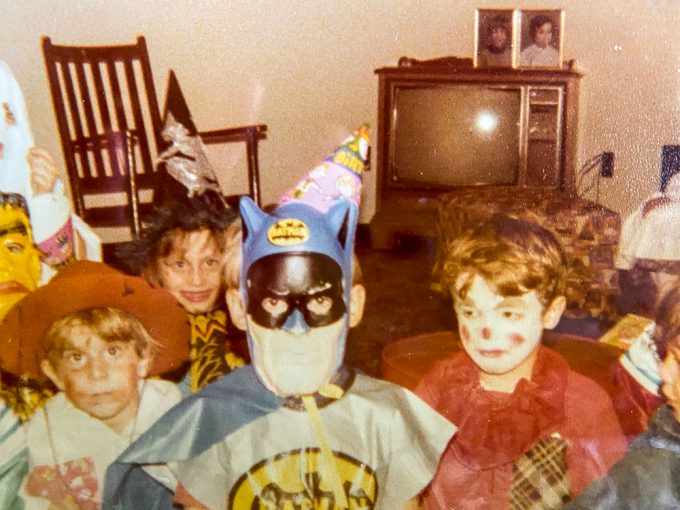The image captures a nostalgic scene likely from the 70s or 80s, with a grainy, orangish or sepia tint. It depicts a children’s birthday party with several kids in costume, possibly on Halloween. In the foreground, the birthday boy is dressed as Batman, identifiable by his black mask, blue ears, Batman symbol on his chest, and a pink cone birthday hat. Beside him, to the right, is a sad-faced clown with white face makeup and red rosy cheeks. Further to the right, partially cut off, is another child whose costume is unclear. To the left of Batman, a cowboy in a poncho and hat stands, face slightly dirty.

In the background, a girl dressed as a witch can be seen, identifiable by her costume's conical hat. Additionally, there's a cut-off view of a child in a Frankenstein mask, and another child's legs covered in bedsheets, resembling a ghost costume. The setting includes a boxy, old-style TV with a glass screen, displaying two framed portraits of a boy and a girl on top. To the left of the TV is a brown rocking chair. The room’s brown carpet adds to the retro ambiance, reinforcing the photograph’s vintage feel. Some children are smiling, while others seem less enthusiastic, portraying a candid moment typical of its era.